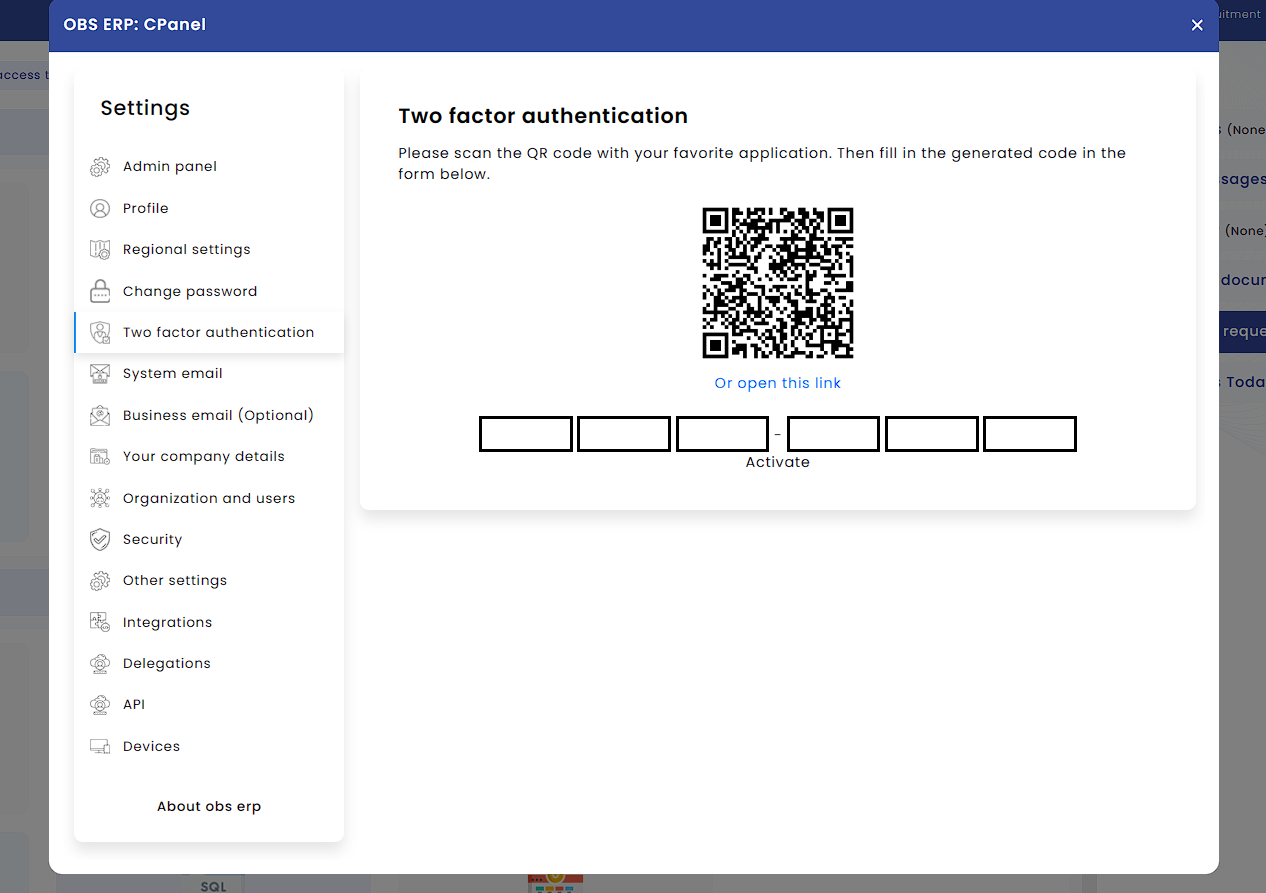This screenshot captures the user interface of the OBS ERP cPanel as displayed on a website. At the top of the page, a blue banner prominently displays the text "OBS ERP: cPanel." In the top right-hand corner of this banner, there is an exit button symbolized by an 'X'.

On the left-hand side, there is a vertical navigation column featuring various settings, each accompanied by an icon. The settings listed are:

1. Admin Panel
2. Profile
3. Regional Settings
4. Change Password
5. Two Factor Authentication (selected)
6. System Email
7. Business Email (optional)
8. Your Company Details
9. Organization and Users
10. Security
11. Other Settings
12. Integrations
13. Delegations
14. API
15. Devices

At the bottom of this list, there is text that reads "About OBS ERP."

On the right-hand side, the interface displays the detail page for the currently selected setting, "Two Factor Authentication." The header "Two Factor Authentication" is followed by instructions for the user: "Please scan the QR code with your favorite application. Then fill in the generated code in the form below."

Immediately below these instructions, a QR code is provided, along with a hyperlink that reads "Open this link." Beneath the link, there are six input boxes where the user is prompted to enter the specific code generated by their authentication application.